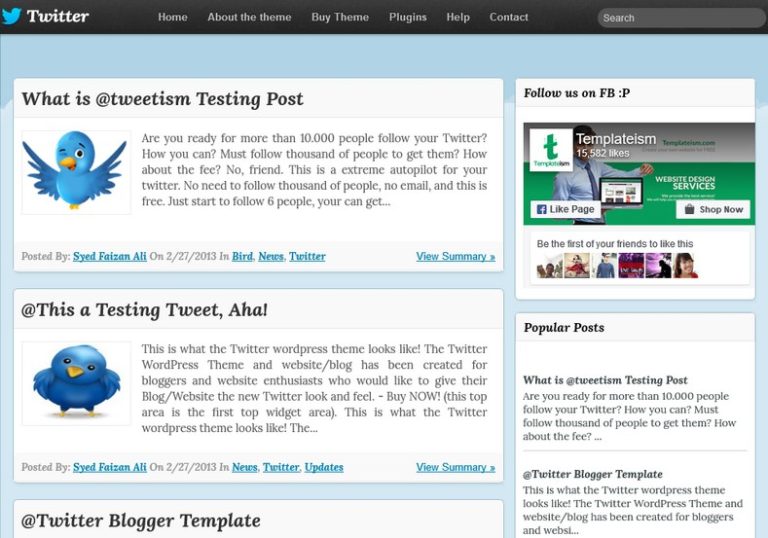This image is a desktop screenshot showcasing a webpage with a Twitter-like aesthetic, but is not Twitter itself. The page features a black header with white text including navigation options: Home, About the Theme, By Theme, Plugins, Help, Contact, and a search box. The centerpiece of the header is the iconic blue bird logo with the text "Twitter."

On the left side of the screen, there is a sidebar housing a cartoonized blue bird and text indicating that a post was submitted by Saeed Faizan Ali on February 27, 2013, categorized under Bird, News, Twitter, and View Summary. The title of the post is, "What is Tweetism? Tweeting Post." The post appears to be an advertisement promising easy Twitter growth without the usual prerequisites of following thousands of users or providing email information. It claims you can gain significant followers by following just a few people.

Below this, there is another post by the same author, dated the same day, listed under News, Twitter, Updates, and View Summary, featuring another blue bird in a different pose. The post is a testing tweet introducing a Twitter WordPress theme designed for bloggers who want to emulate Twitter's look on their site. The post encourages users to purchase the theme and highlights that the top area is the first widget area of the theme.

The snippet of the next headline reads, "At Twitter Blogger Template," but is cut off. On the right side of the screen, there is a section indicating that users can follow the source on Facebook, with the name "Templateism" displayed in green lowercase. This entity has 15,582 likes on Facebook, with options to like the page and shop now.

The "Popular Posts" section repeats the two featured posts, suggesting they are the most engaging content available. Overall, the webpage is clearly an advertisement for a Twitter-themed WordPress layout or tool aimed at Twitter enthusiasts and bloggers.